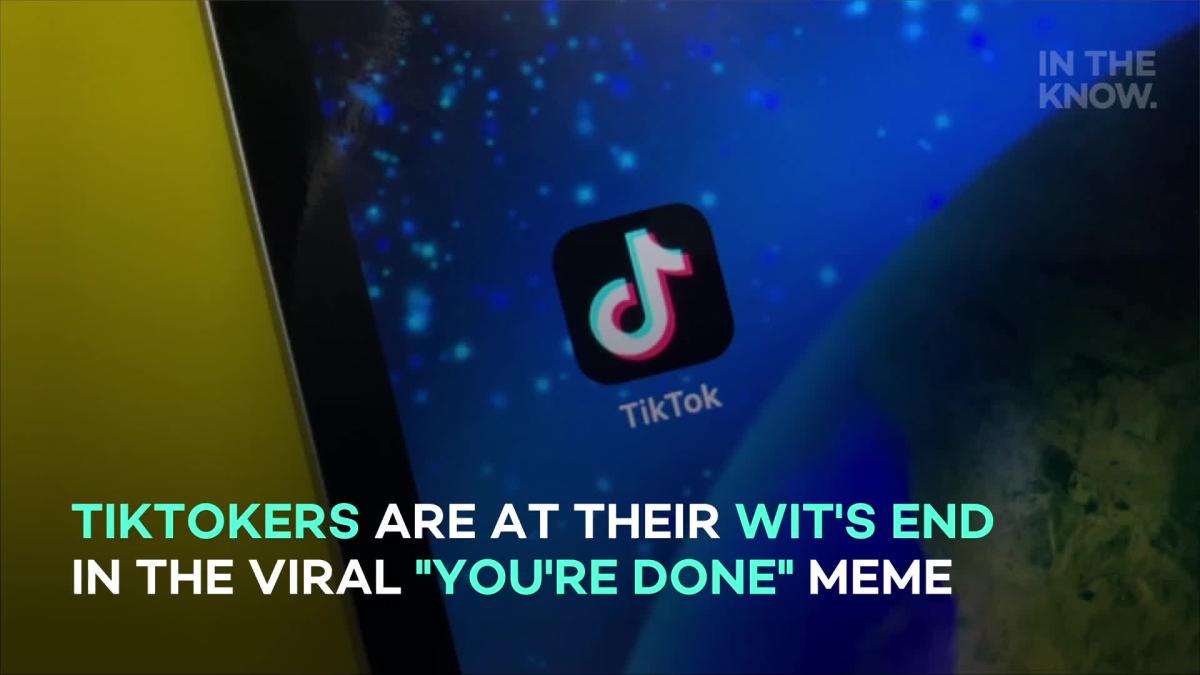This promotional image for an app or website prominently features the TikTok icon in the center. The icon is displayed within a black square and consists of the white TikTok logo outlined in a vibrant purple and green border. Below the icon, the text "TikTok" is written in white capitals, T-I-K-T-O-K. 

In the upper right-hand corner, there's faint gray text that reads "in the know" with the phrase "in the" followed by "K-N-O-W" and a small period. The bottom right-hand corner of the image features a globe graphic set against a blue starry sky, which appears to be displayed on a tablet screen. This is indicated by the thin black border on the left side of the globe, suggesting the screen's edge.

The text "TikTokers are at their wits' end in the viral 'you're done' meme" is written in a bluish-green font against an olive green background located on the left side of the image. The overall design elements are arranged to convey a sense of urgency and trendiness surrounding the "you're done" meme on TikTok.